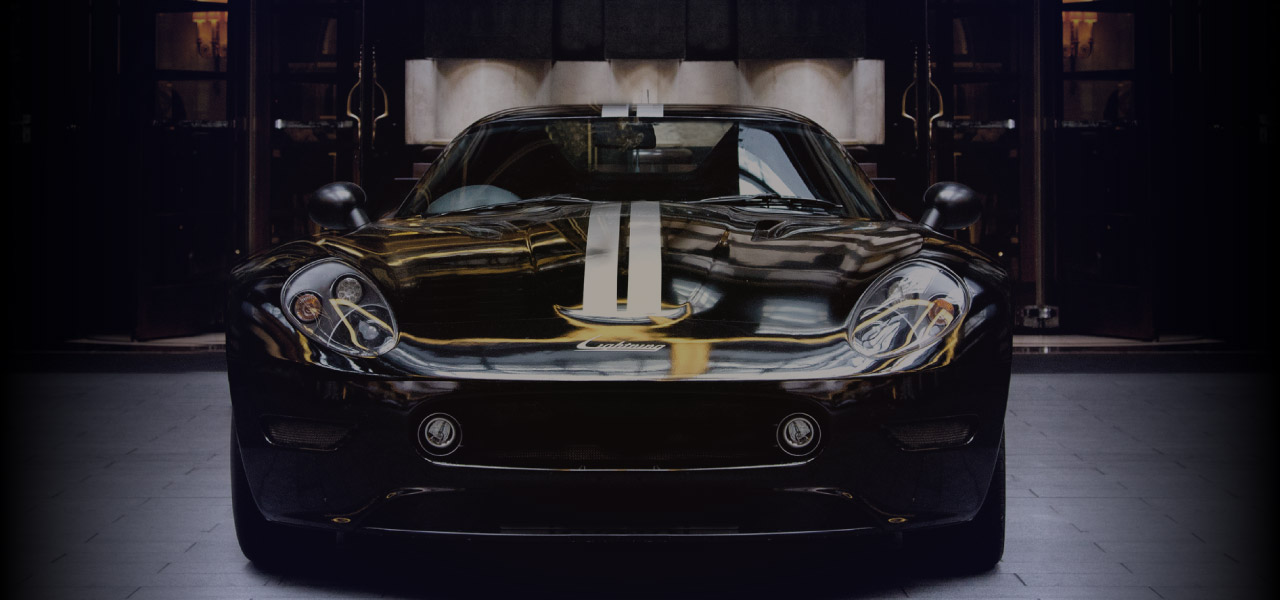This image captures an artistic and moody photograph of a sleek, shiny black sports car reminiscent of a Dodge Viper. The car is photographed head-on, emphasizing its elegant and menacing front appearance, with headlights and fog lights that resemble the predatory eyes of a viper. The central focus is on the car's hood, adorned by two metallic steel gray stripes running down the middle. The car is set against a dark, sombre background with dark gray tiles and black curtains, possibly situated in a dimly lit garage or showroom. The lack of bright lighting adds to the dramatic and classy feel of the scene, reflecting golden hues off the car’s polished surface. Despite the elusive branding details, the image highlights the car’s striking design, with a script barely visible just below the stripes, enhancing its mysterious and high-end allure.